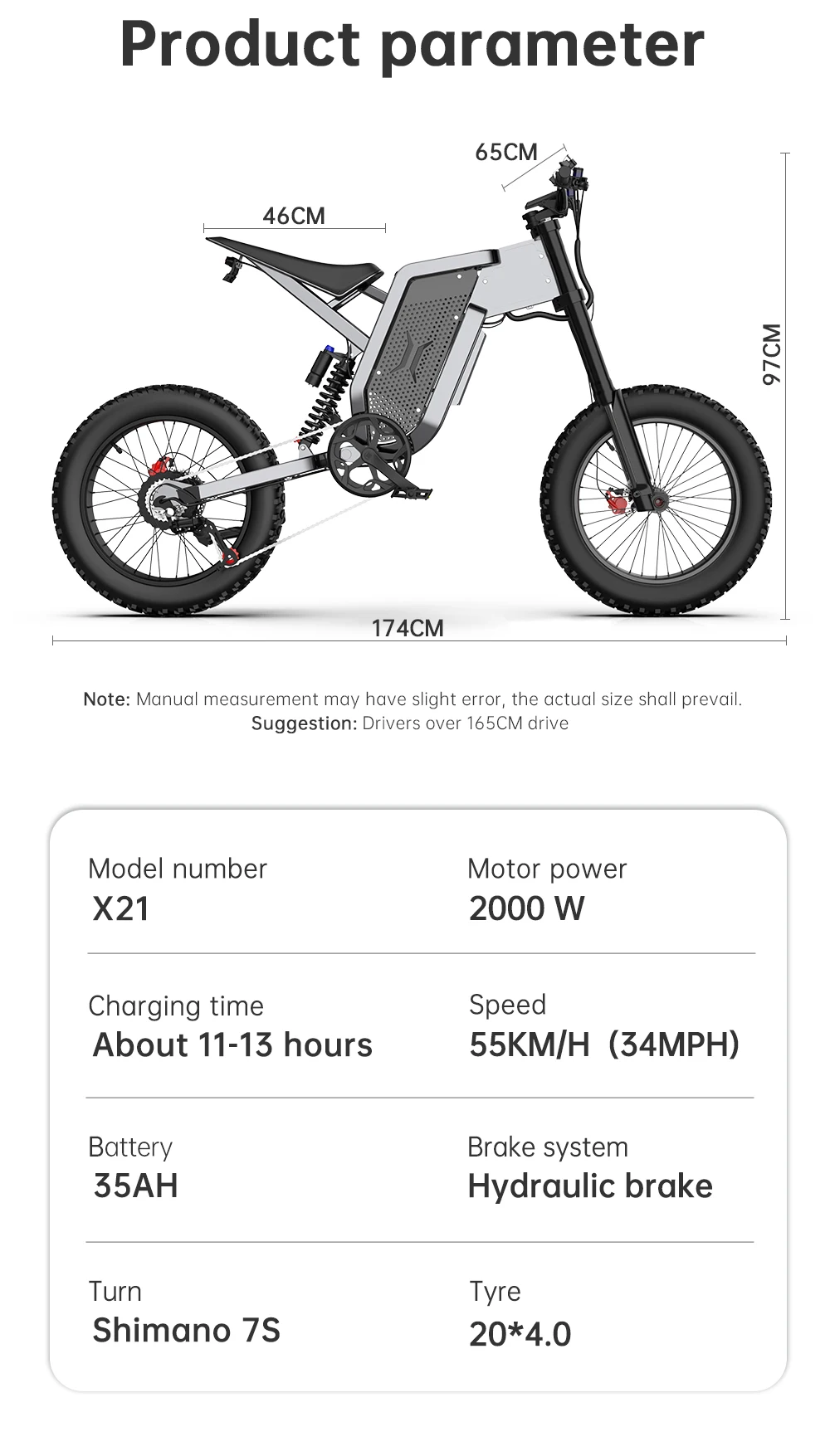This image is a detailed screenshot in portrait mode, primarily displaying the specifications of a motorized bicycle under the heading "Product Parameter" at the top center in black text. Below the heading is a visual representation of the bicycle along with its various measurements. 

The dimensions are as follows:
- The length from the rear tire to the front tire is 174 centimeters.
- The height from the bottom of the tire to the top of the handlebar is 97 centimeters.
- The handlebar width spans 65 centimeters.
- The seat height measures 46 centimeters.

A note beneath the measurements indicates that manual measurement may have slight errors and emphasizes that actual sizes may vary. It also suggests that the bicycle is suitable for drivers over 165 centimeters tall, raising a question about whether the units specified are centimeters or not.

Additionally, enclosed within a rounded rectangle, there are further technical details:
- Model Number: X21
- Motor Power: 2,000 watts
- Charging Time: Approximately 11 to 13 hours
- Top Speed: 55 kilometers per hour (which converts to 34 miles per hour)
- Battery Capacity: 35 Ampere-hours (AH)
- Brake System: Hydraulic brake
- Gear Shift: Shimano 7-speed system (Shimano 7S)
- Tire Size: 20 x 4.0 inches, with "tire" spelled as "TYRE"

These detailed specifications paint a comprehensive picture of the motorized bicycle, though there is some ambiguity regarding the measurement units.